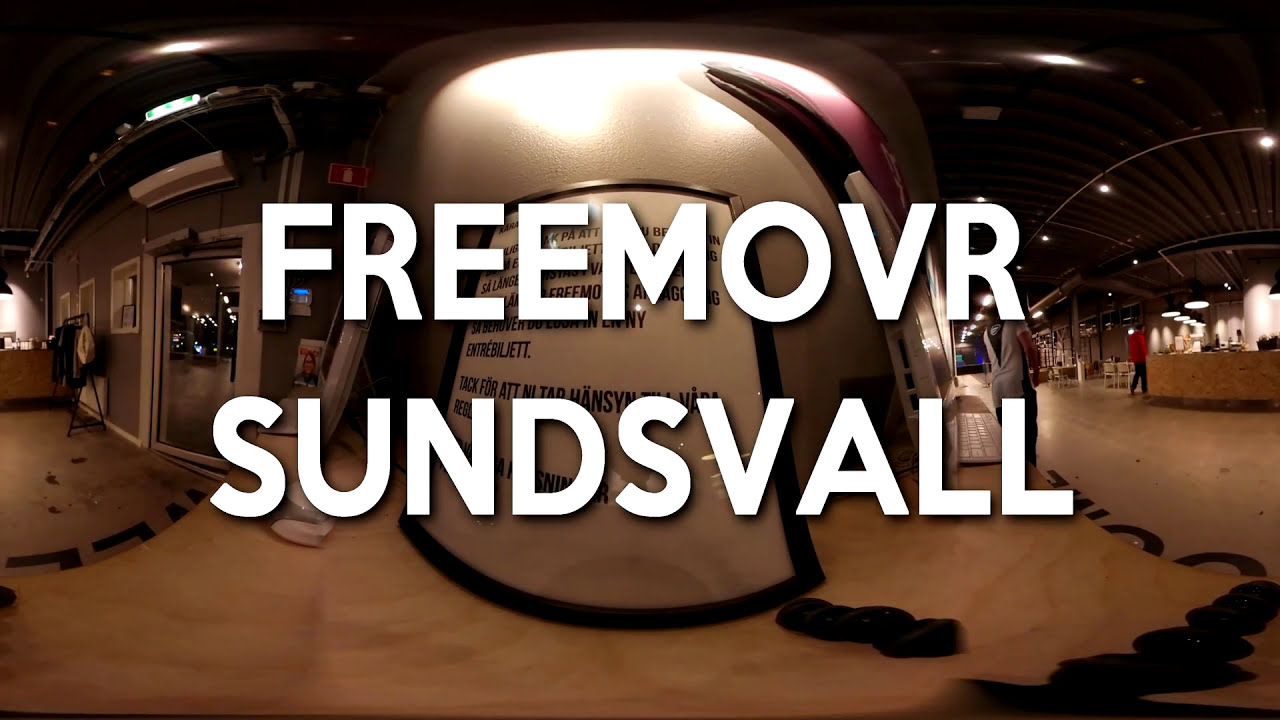This detailed photograph captures the interior of a bustling, indoor shopping area or mall. Central to the image is a prominent sign with bold, white letters displaying "F-R-E-E-M-O-V-R-S-U-N-D-S-V-A-L-L," likely a phrase in a foreign language. Surrounding the sign, the setting includes a mixture of hard-surfaced floors, doorways, and windows on the left, all illuminated by ceiling lights and lamps. 

To the right, a counter with various white items is positioned. Near this counter, a man dressed in a long-sleeve red shirt and darker pants stands, while another individual in a white outfit is nearby. Scattered throughout the space are kiosks and desks, contributing to the busy atmosphere. 

Lastly, the palette of colors ranges from white, black, yellow, maroon, gray, tan, and blue to red, enhancing the diverse and lively indoor environment. With people walking around and engaging with the space, the photograph captures a vibrant scene full of activity, seemingly indicating an ongoing event or convention.